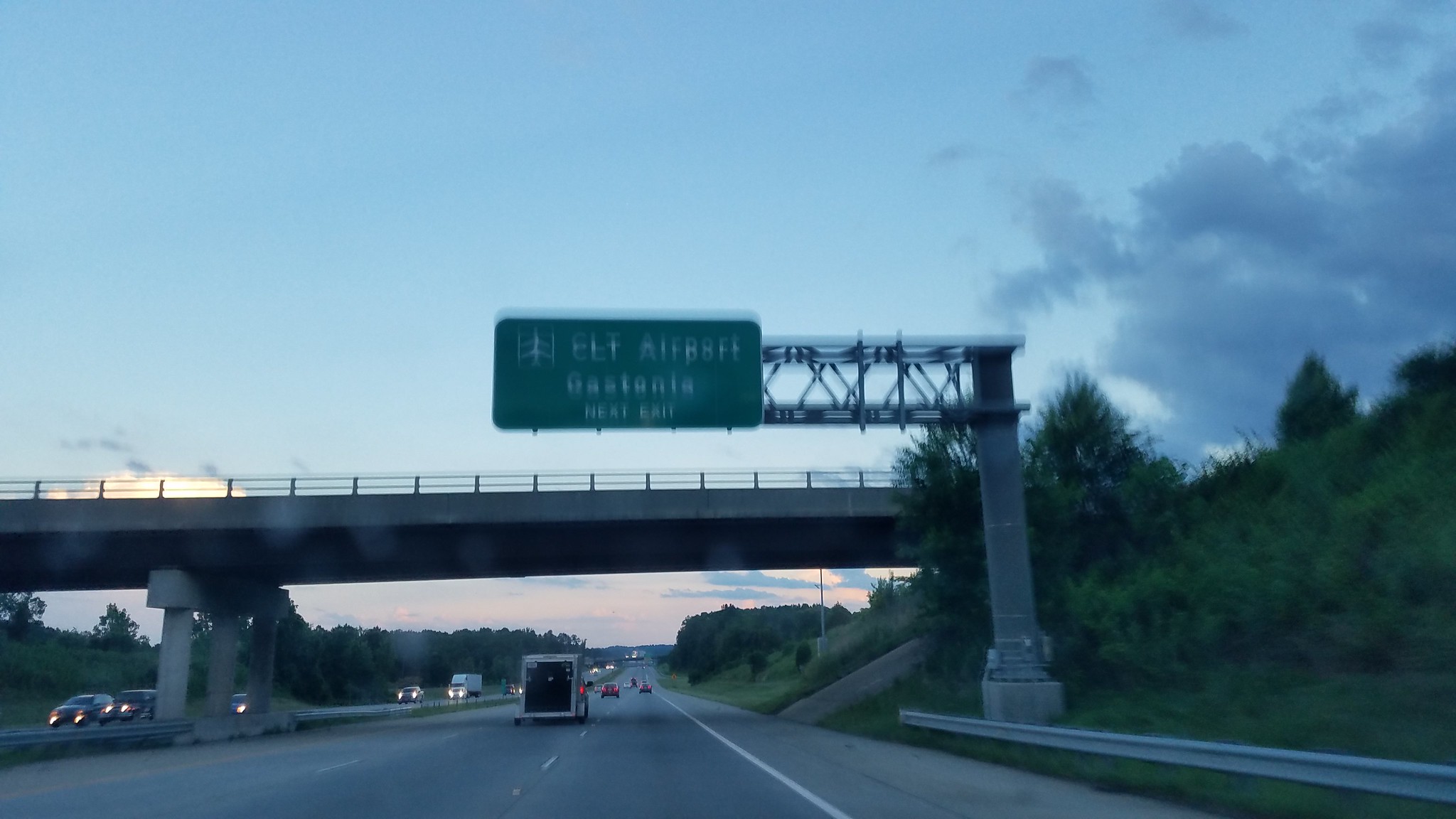This photograph depicts a bustling highway at dusk, captured from the vantage point of a front windshield. The six-lane road is teeming with moderate traffic, as vehicles move steadily under the dimming sky. The encroaching darkness has prompted drivers to turn on their headlights, casting a glow across the asphalt. Dominating the scene is a bridge or overpass, stretching horizontally across the frame.

Above the road, a green rectangular overhead sign is illuminated, though slightly blurred and doubled in the image. The sign contains multiple inscriptions: "ELT Airport," "Gastonia," and "Next Exit," with a partial depiction of an airplane to indicate airport directions. There is some ambiguity around the letters "ELT," which could possibly read "CLT" due to the blur.

Accentuating the dynamic nature of this highway snapshot, an open-back U-Haul truck is visible in the adjacent lane, adding to the sense of movement and everyday activity on this evening commute.